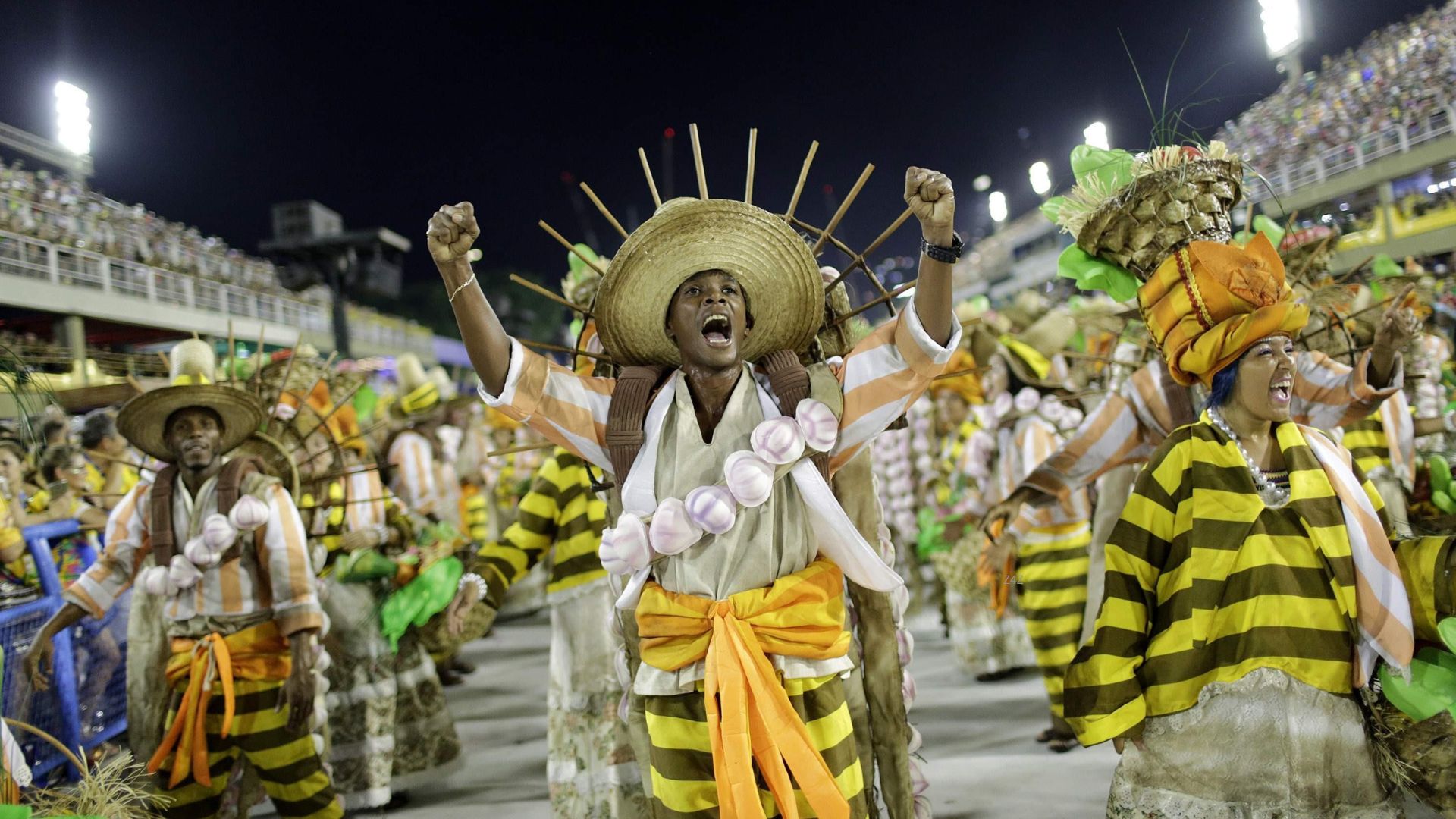The image captures a vibrant festival taking place in a bustling stadium in Atlanta, characterized by large permanent bleacher seating and towering spotlights typical of sporting events. The event appears to be a parade, overflowing with colorful and festive energy. Central in the photo is a jubilant figure, possibly male, with arms raised and mouth open in an expression of victory or celebration, wearing an elaborate straw hat adorned with lollipop-like decorations. This figure, along with other participants, sports distinctive costumes featuring yellow and brown (or orange) bumblebee-like stripes. These outfits consist of either pants or shirts, coupled with decorative sashes possibly resembling strings of garlic, suggesting an agricultural or harvest theme. The woman to his right contrasts with a long white skirt paired with a striped shirt, and balances a basket piled with fruits or vegetables atop her hat. The celebratory attire of all attendees includes wide-brimmed, decorated hats and various sashes or wraps, adding to the vivid display. The crowd, predominantly composed of African Americans, marches joyfully through the stadium, applauded by rows of engaged spectators. This captures the essence of a deeply rooted cultural tradition or festive celebration, marked by spirited dancing, marching, and communal joy.